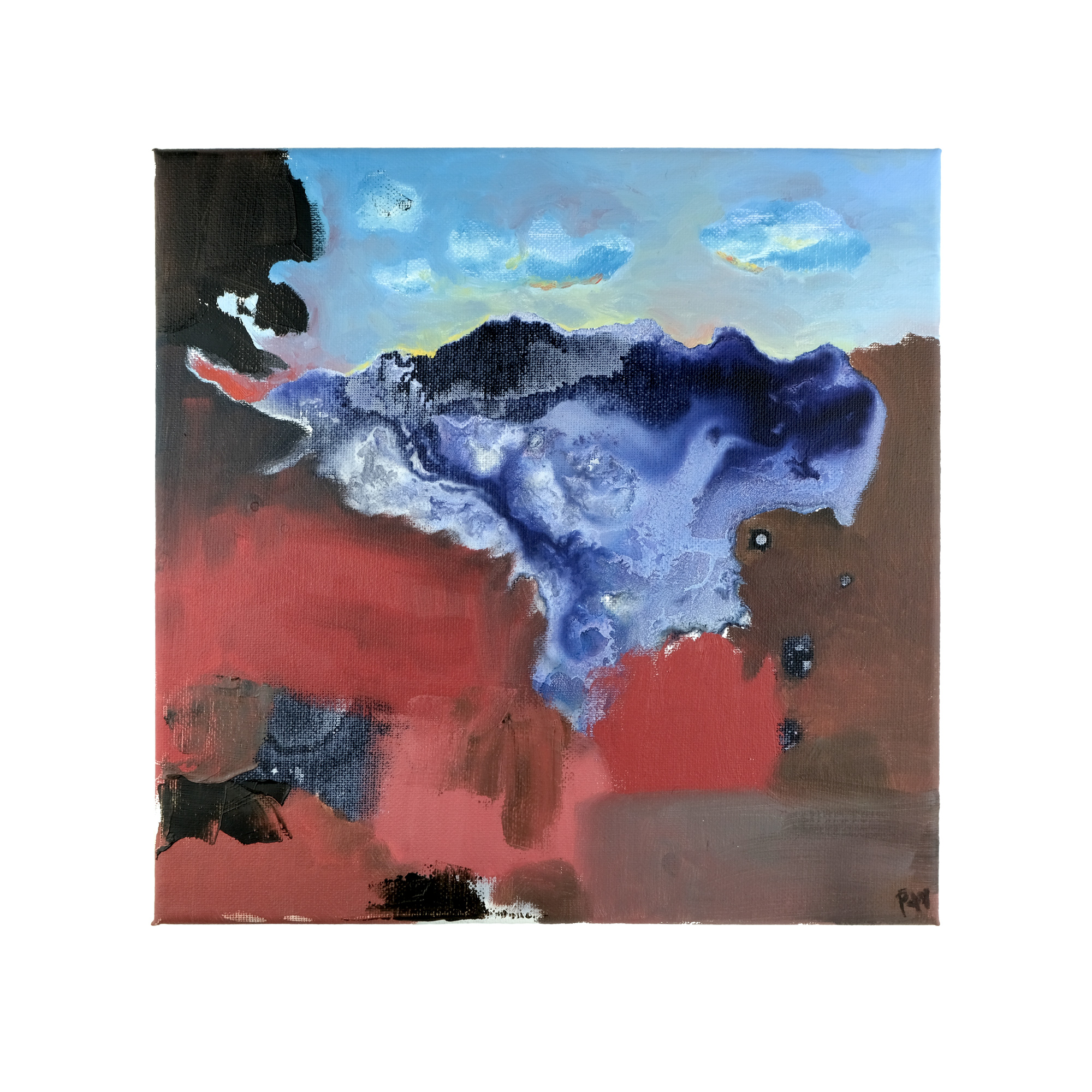An abstract oil painting on canvas features a blend of vibrant and earthy tones. The composition transitions from a light blue and white sky with scattered clouds at the top to deeper shades of blue, resembling water, dominating the central area. On the left side, dark hues possibly represent a tree with some dark brown patches below, potentially indicating roots. The right-hand side has a prominent area of brown and red, giving the impression of a dirt road or earthy surface. The painting integrates blotches of red, blue, brown, black, and gray, creating a dynamic yet unclear landscape that evokes emotion rather than depicting a specific scene. The texture and color transitions, including a notable marble effect in the blues, add depth and intrigue. In the corner, partially legible initials, possibly "P-A-V," mark the artist's signature. This piece exudes an emotive aesthetic, perfect for home decor, despite its abstract and non-photorealistic nature.